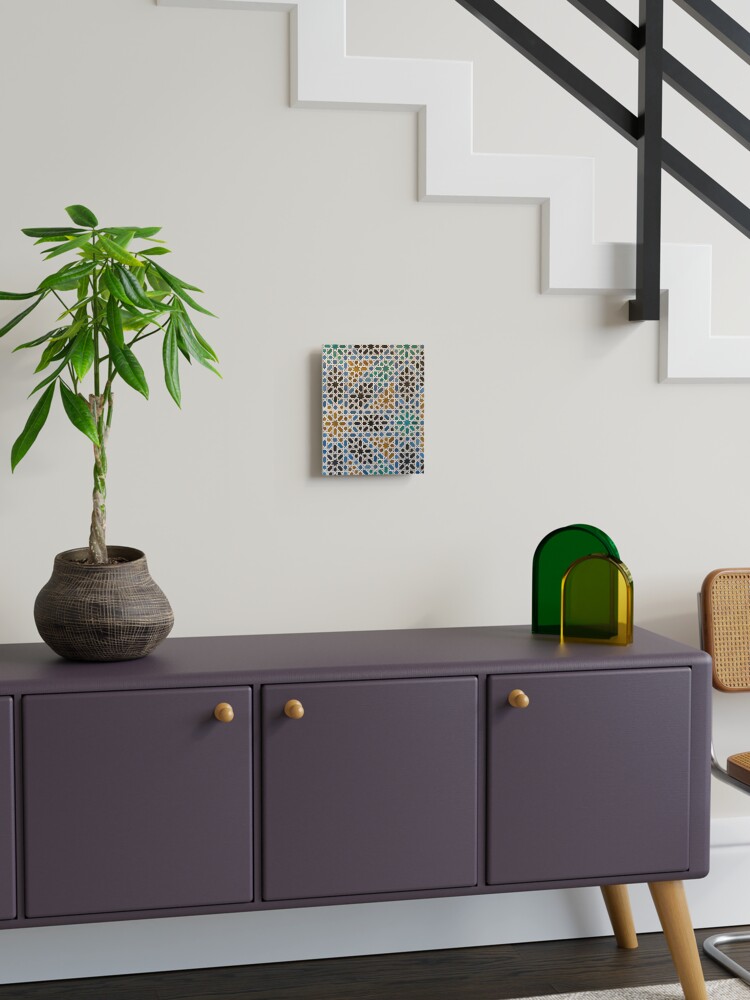The image depicts a modern mid-century console table or cabinet, painted in a muted purple shade with an interesting leather-like finish. Positioned against a white wall and in front of a staircase with black railings and wooden steps, the table stands on a brown wooden floor. The table has visible legs on the right side and features light tan wooden knobs on its drawers. On the left side of the table, there is a wicker vase containing a plant with a long stalk and green leaves. To the right of the table, a few green and yellow transparent objects are placed. Hanging directly above the console table is a colorful piece of graphic artwork. Adjacent to the table on the right side of the image is a brown chair, and a portion of a stairway carpet or rug is visible near one of the table's legs, further accentuating the modern aesthetic of the room.